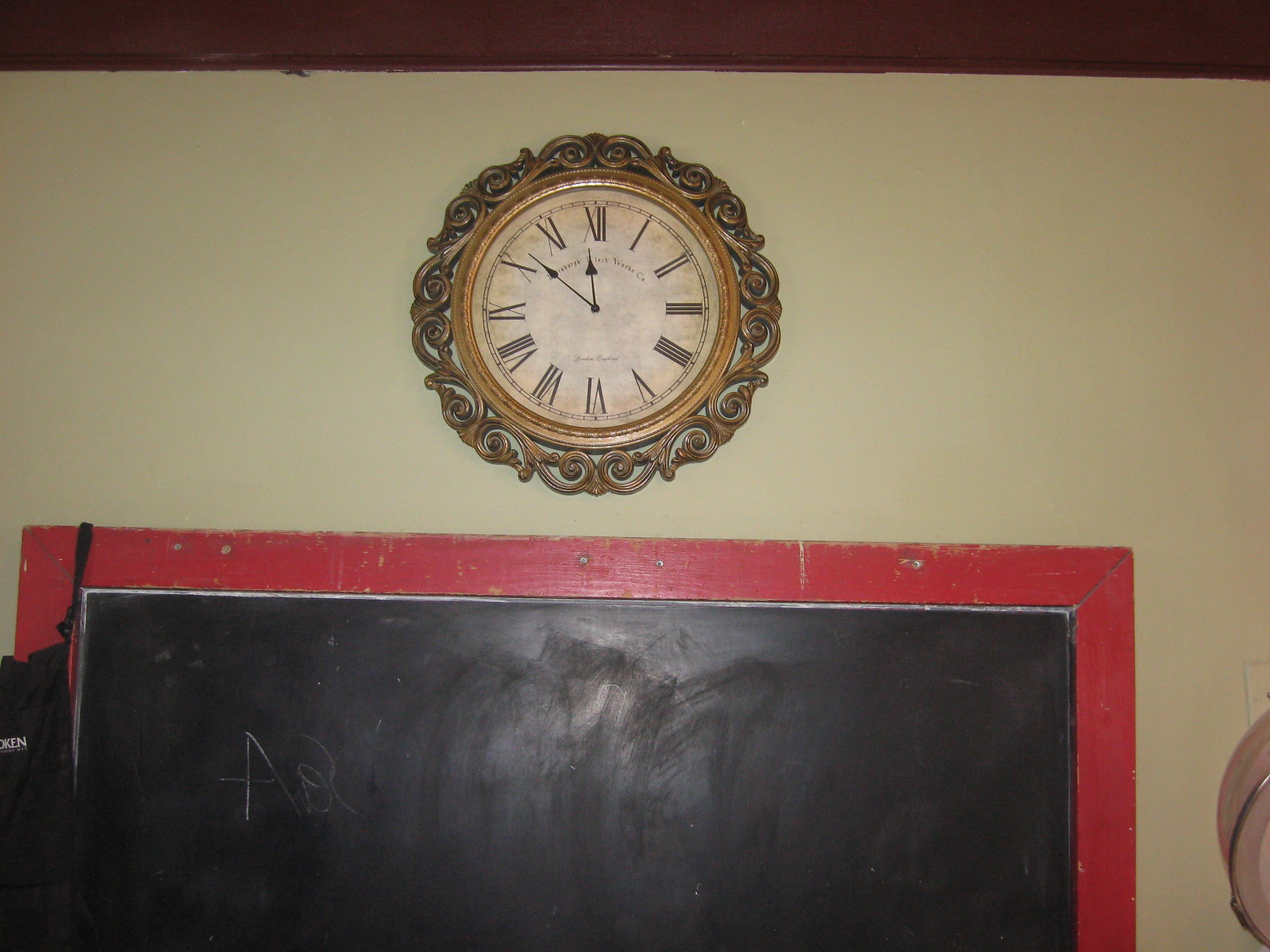The image displays a room with a yellowish beige plaster wall featuring a prominent, ornate wall clock and an aged chalkboard beneath it. The clock, positioned in the middle top of the wall, has a round face with black Roman numerals and old-fashioned black hour and minute hands, showing the time at seven minutes to twelve. The clock's face is off-white with tan spots, enclosed by a yellow bronze outline adorned with intricate floral and spiral wooden carvings. Below the clock, embedded into the wall, is a blackboard framed by a worn, distressed red wooden border, approximately five centimeters wide. The chalkboard has some white writing scribbled in the top left corner. The overall image, though not in sharp focus, clearly captures these elements in the color photograph.